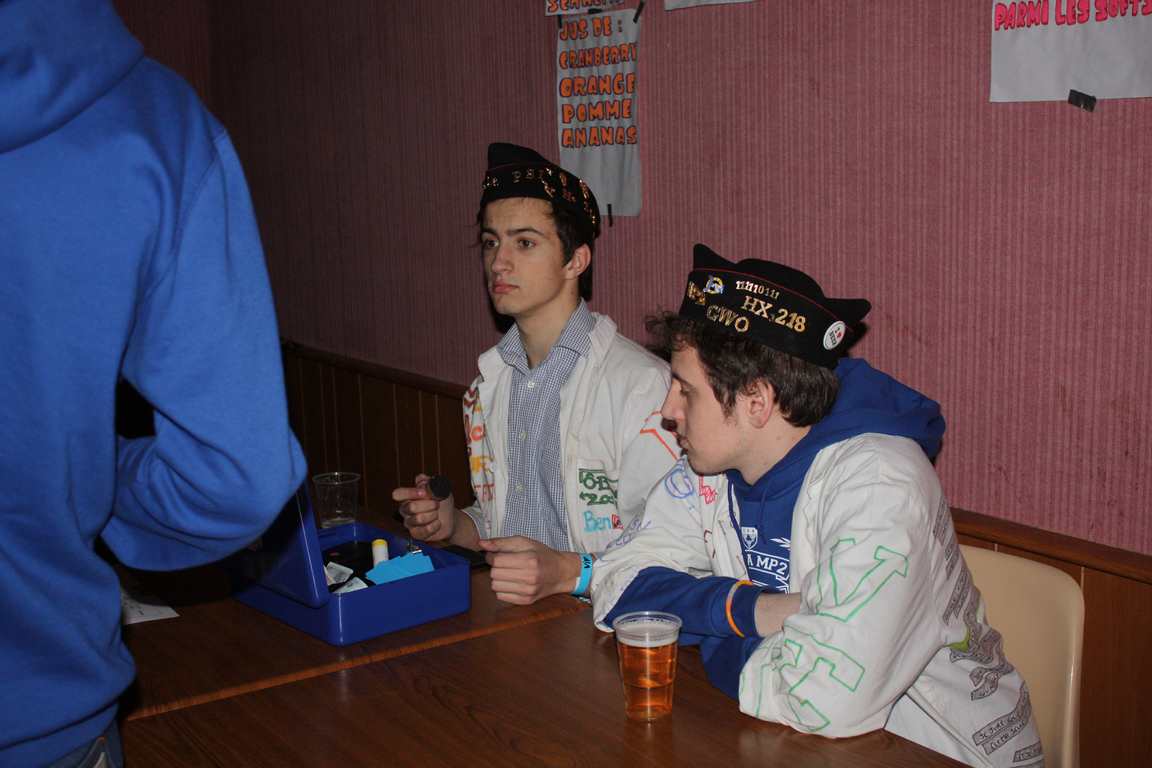The photograph captures an indoor scene featuring three individuals. On the left, only the backside of a person dressed in a light blue hoodie is partially visible from the right waist up to the shoulder, with their arm bent at a 90-degree angle. Dominating the right side of the image are two young men, possibly in their late teens or early twenties, seated at a brown table with a wood grain pattern. They appear to be in some kind of uniform, consisting of white and yellow overcoats with custom writing, reminiscent of ceremonial or club attire, and black military-style hats with gold lettering, including "HX," "218," and "GWO."

One of the young men, with dark hair, is wearing a white jacket over a blue hoodie and holds a glass of beer, identifiable by the foam at the top. In front of him is an open blue box, likely for collecting payments. His companion, similarly dressed in a white jacket over a blue and white collared shirt, is holding a stamp in his right hand, suggesting they are involved in ticketing or fee collection. The background features a pinkish-red wall adorned with posters in French, one of which has orange lettering while another has blue with red lettering.